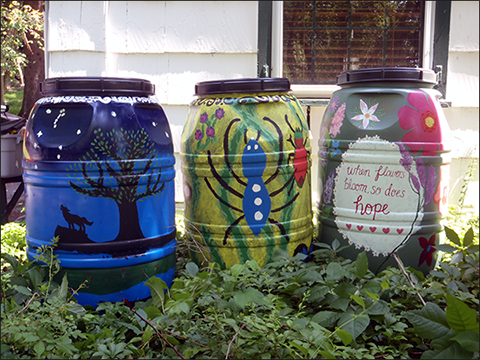The image showcases three large, hand-painted rain barrels positioned against a house with white paneled siding and a brick wall. Each barrel features a black twist-off lid and is surrounded by green plants at their base. The barrels vary in designs: the leftmost one illustrates a nighttime scene with a dark blue sky, white stars, a tree, and a wolf howling at the moon; the middle depicts a blue insect with white dots for eyes and on its back, crawling among purple flowers and grass; the rightmost barrel is adorned with colorful pink, white, and purple flowers and a white ball, accompanied by the poem "When flowers bloom, so does hope." The entire composition suggests a whimsical garden setting, adding a touch of artistic charm to functional objects.